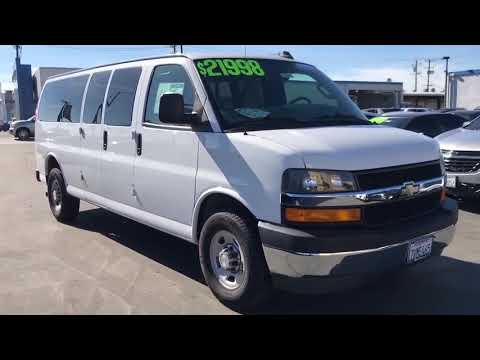The photograph captures a white Chevrolet work van, positioned in a parking lot, likely at a car dealership. The vehicle is angled towards the front right corner, revealing its right-hand side, which includes a passenger door and a sliding door behind it. The van features four windows along its side: one on the passenger door and three additional windows towards the back. Noteworthy details include black tires with white inner rims, a black fender, and a silver grille. An orange light is situated near the lower front end, and a license plate with indiscernible numbers is affixed to the front. The windshield displays a bright green price tag reading $21,998, prominently positioned in the upper left-hand corner. The background shows several other cars lined up, some also bearing price tags, reinforcing the dealership setting. The scene is illuminated by sunlight, under a blue sky with visible distant buildings, while the parking lot's pavement is a faded gray asphalt.